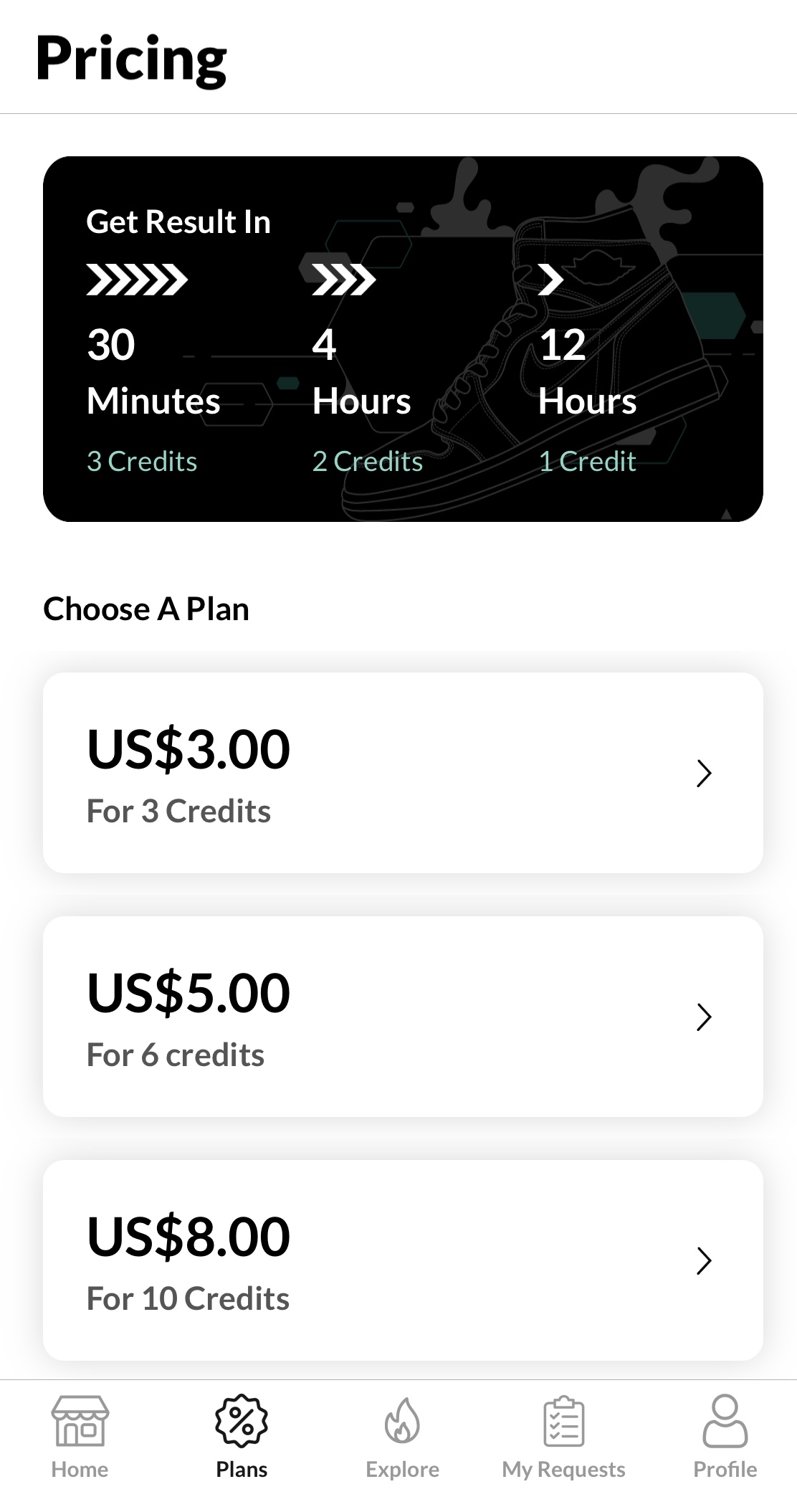This image captures the pricing page of a website displayed on a smartphone screen. The focal point of the background is a sleek, black box featuring an image of a Nike high-top sneaker. Above this image, the text "Get result in" is prominently displayed in white. Below this phrase, a sequence of five vertical right-facing arrows leads to the text "30 minutes, three credits." Moving rightward, a trio of horizontal right-facing arrows are aligned with the text "4 hours, two credits," and further to the right, a single right-facing arrow is positioned above the text "12 hours, one credit."

Furthermore, beneath this set, a section labeled "Tuesday Plan" showcases three distinct boxes displaying credit options. The first box reads, "US $3 for 3 credits," accompanied by a right-facing arrow to its right. The second option states, "US $5 for 6 credits," also with a right-facing arrow beside it, and the third box displays, "US $8 for 10 credits," with the same right-facing arrow to its right.

At the bottom of the page, a navigation bar features five icons: a home icon, a plans icon (highlighted to indicate the current page), an explore icon, a my requests icon, and a profile icon.